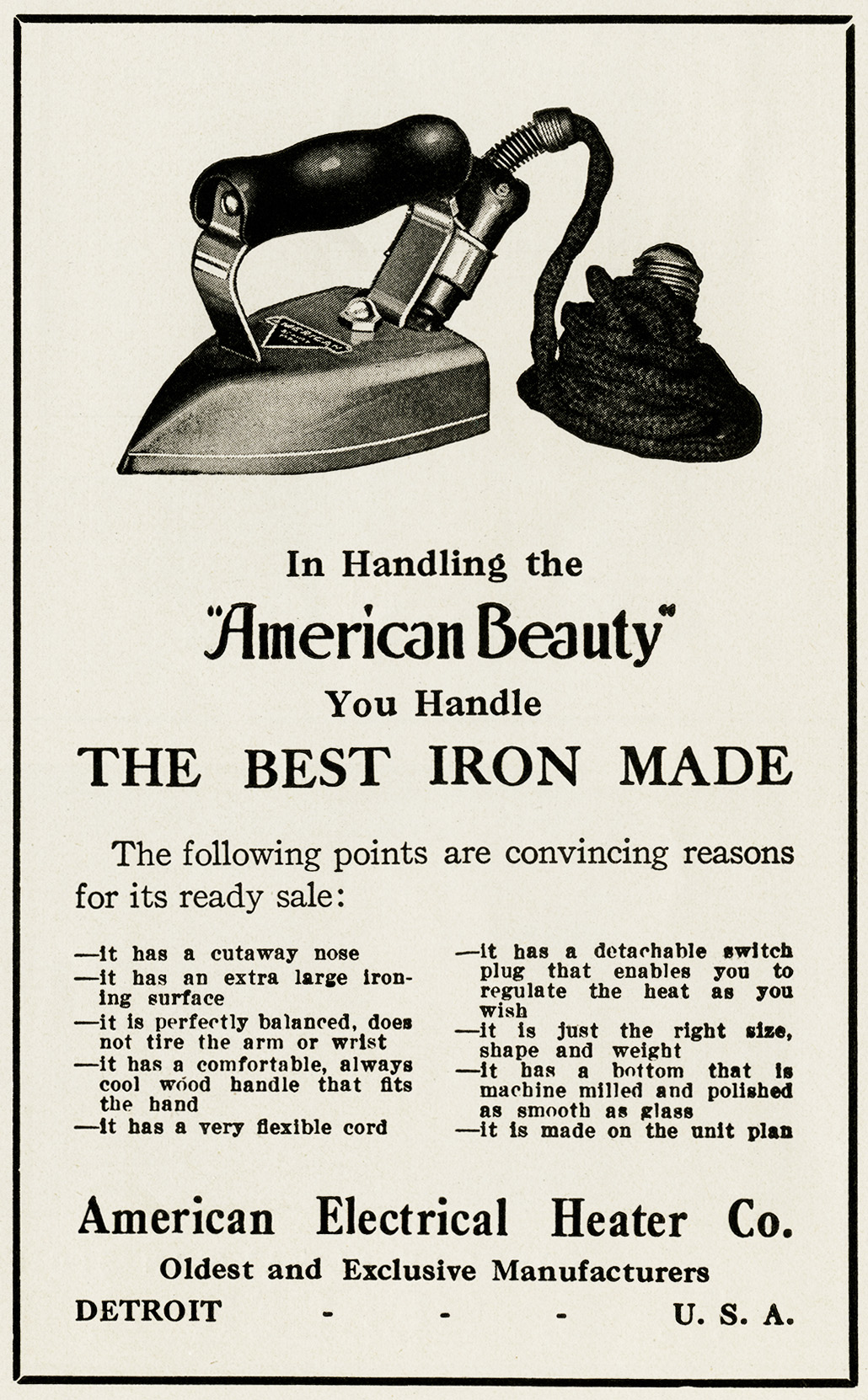This black-and-white newspaper advertisement from the early 1900s features a detailed illustration of an old-fashioned electric iron centered at the top. The iron, described as the "American Beauty," has a triangular base, a cool-to-touch wooden handle, and a flexible attached cord. Its meticulously designed form resembles an upside-down boat with a polished, glass-smooth bottom, and it boasts a perfectly balanced structure that prevents arm or wrist fatigue.

The advertisement claims, “In handling the American Beauty, you handle the best iron made.” It provides multiple convincing points for its superior quality, including a cutaway nose, an extra-large ironing surface, and a detachable switch plug for heat regulation. Additionally, it emphasizes that the iron is "just the right size, shape, and weight," and is constructed on the unit plan.

The bottom of the ad features the manufacturer's details, proclaiming the American Electrical Heater Co. as the oldest and exclusive manufacturer based in Detroit, USA. The ad is bordered by a black line and set against a light gray or cream-colored newsprint background, capturing the essence of early 20th-century advertising with its focus on functional merit over aesthetic appeal.